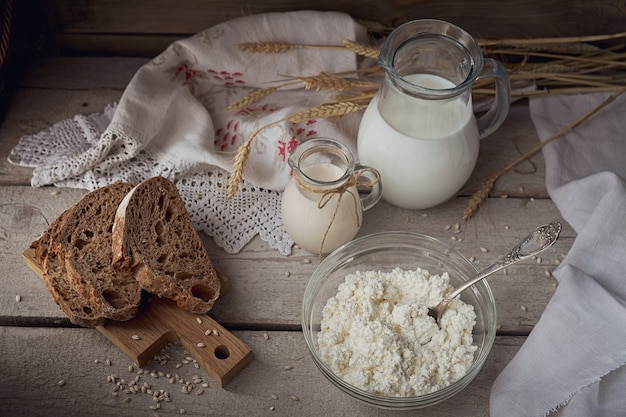In the photo, there is a rustic scene set upon a light brown or grayish wooden table with long, unfinished wooden planks stretching horizontally, reminiscent of an outdoor picnic setting. On the left side of the image, there's a small, wooden cutting board with three to four slices of dark, whole wheat bread adorned with white seeds. Beside the bread, there's a clear bowl containing a thick, white substance, possibly rice, with a silver fork or spoon sticking out.

Toward the back, there's a clear pitcher filled with white milk, accompanied by a smaller clear pitcher tied with tan twine, containing a creamy or tan-colored liquid. Spread across the scene are stalks of tan wheat, with their stems providing a rustic feel. The table is decorated with a white tablecloth featuring red elements, likely representing grapes or strawberries with green leaves or stems. Additionally, another white cloth with a bristly edge is placed at the bottom right, enhancing the textured layers of this cozy, pastoral arrangement.